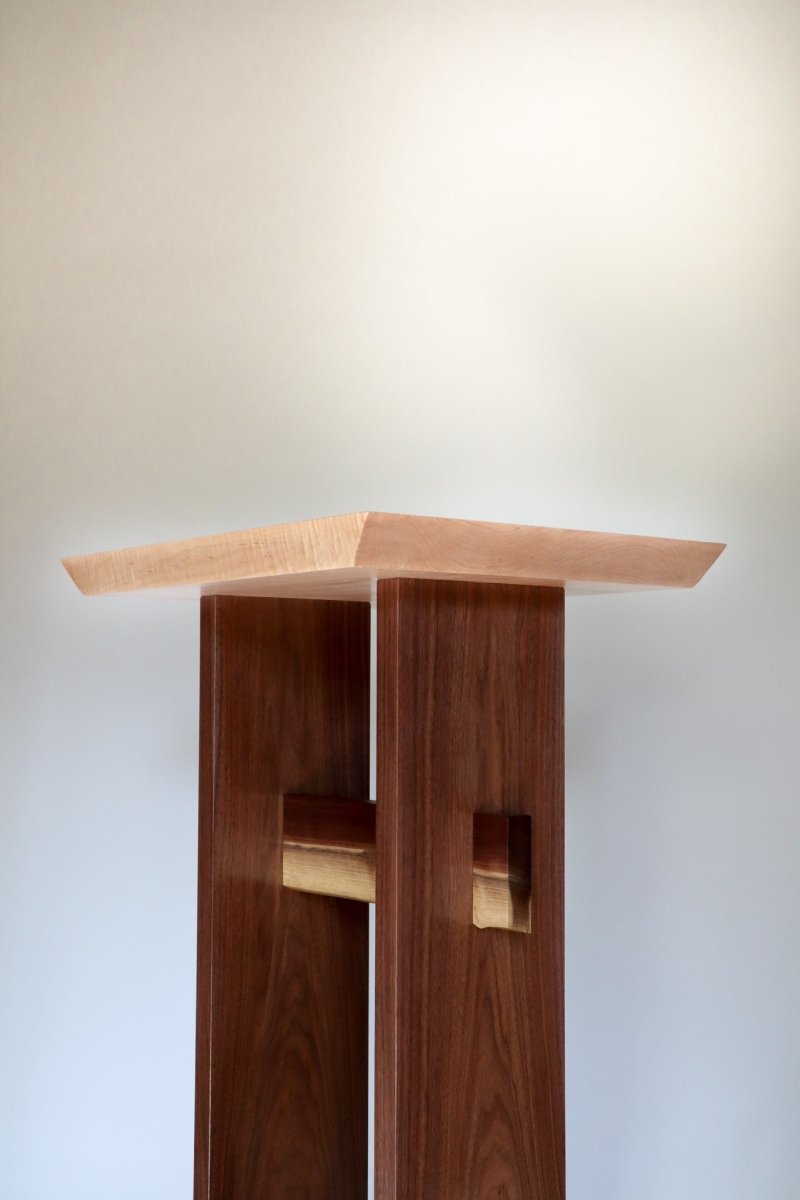The image is a vertically oriented color photograph that features a simple wood platform. The background is a mottled gray with light blue undertones near the bottom and light gray near the top, where a flash creates a light aura in the upper right corner. Centrally positioned in the photograph, extending upward from the bottom middle, are two dark brown vertical wood planks, stained dark brown, creating a stand-like structure. Each plank features a vertically oriented rectangular hole about a third of the way down, through which a light brown wood dowel connects both planks. The dowel is two-toned, darker on top and lighter on the bottom. At the top of these vertical planks, a square beige wood platform with beveled edges is attached, angled with its corner facing the viewer. This tray-like feature binds the two vertical planks at the top, though it is unclear whether it is made of wood or plastic. The overall style of the photograph is realistic, representing the subject clearly and in detail.